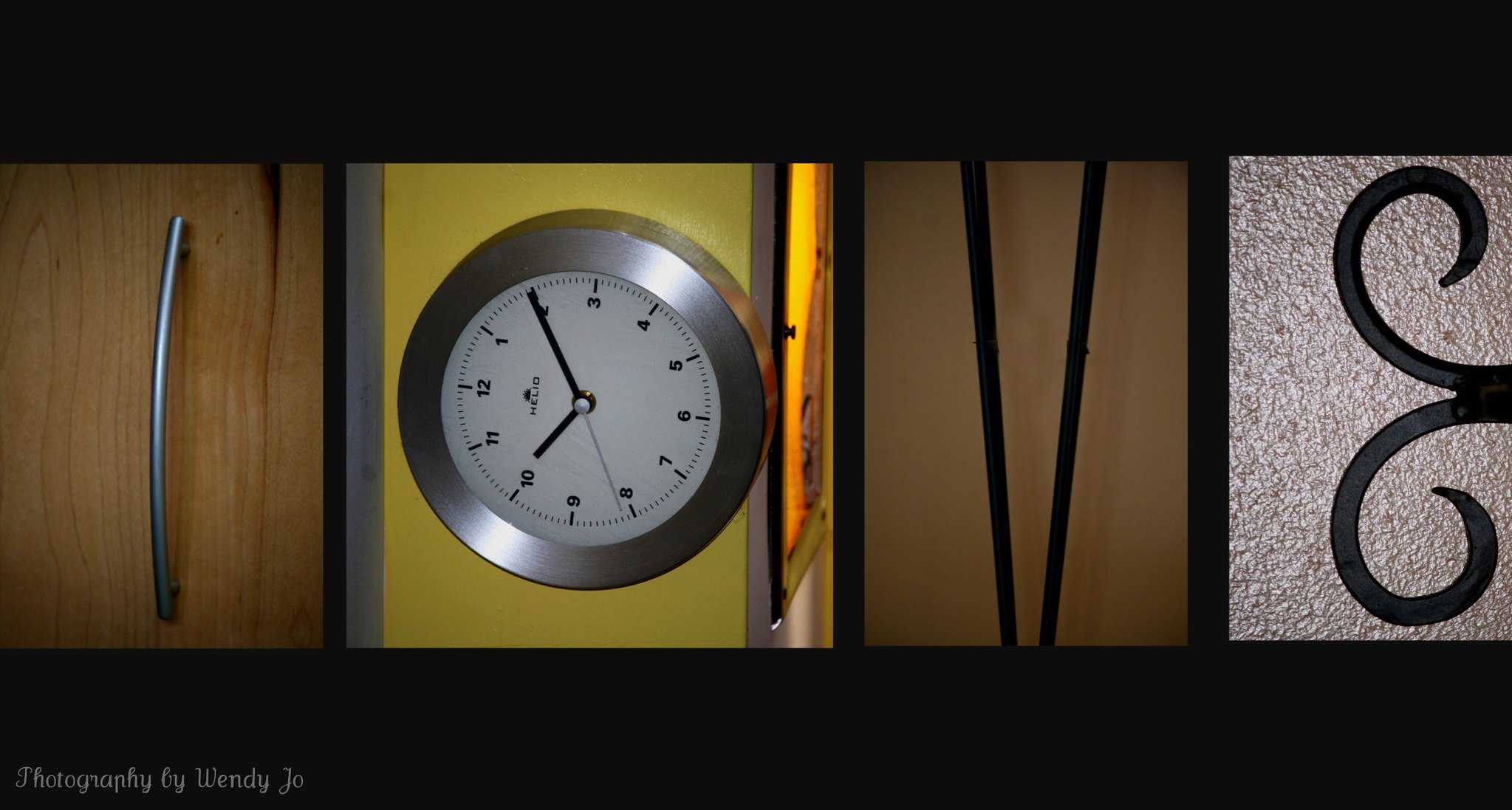This is a photograph that appears rotated 90 degrees, showing a creatively composed word "LOVE" made from various elements. The first element is a sideways-mounted wall clock, with its 12 o'clock pointing left. The clock features a thick silver housing, a white face with small black numbers, and additional lines marking each number and minute. The hands are black, with the second hand being white, and it displays 10:10. This clock forms the letter "O" in the word "LOVE". 

Adjacent to it on a wooden panel is a curved drawer handle turned vertically, resembling the letter "l". Another panel shows intricate metal inlays on wood, slightly angled to form the letter "V". The final element is a decorative metal gate with black horizontal strips and wrought iron curves, forming an abstract "E". 

In the bottom corner, there is a mention of "Photography by Wendy Zhou".